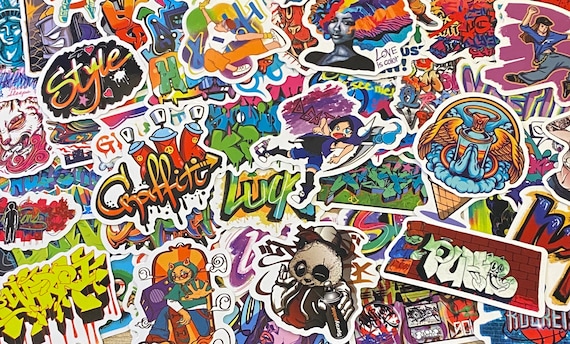The image is a vibrant, animated collage in landscape orientation, densely covered with an eclectic mix of overlapping stickers and artworks. Each element is outlined in white against a neon-colored backdrop, creating a chaotic yet visually rich tapestry. Dominating the scene are various depictions, including a black-and-white zombie panda in the foreground, and anthropomorphic figures like a skateboarder and a woman with a riotously colorful Afro resembling a clown wig. A boombox-wielding character with yellow and orange hair stands out among the eclectic mix, alongside a vertically arranged Bride of Frankenstein-like figure in neon colors.

Random graffiti stickers featuring bubble writing and dripping blood are scattered throughout, some partially obscuring others. Prominent words like "graffiti," "lug," and "style" appear in bold, graffiti-style fonts. Characters and motifs span various themes—from love and harmony to anarchic and punk sensibilities—with images of the Statue of Liberty and an anime-like character in blue and black adding to the diversity. The overall palette is a cacophony of greens, reds, purples, and pinks, making for a striking and unmistakably vibrant scene.